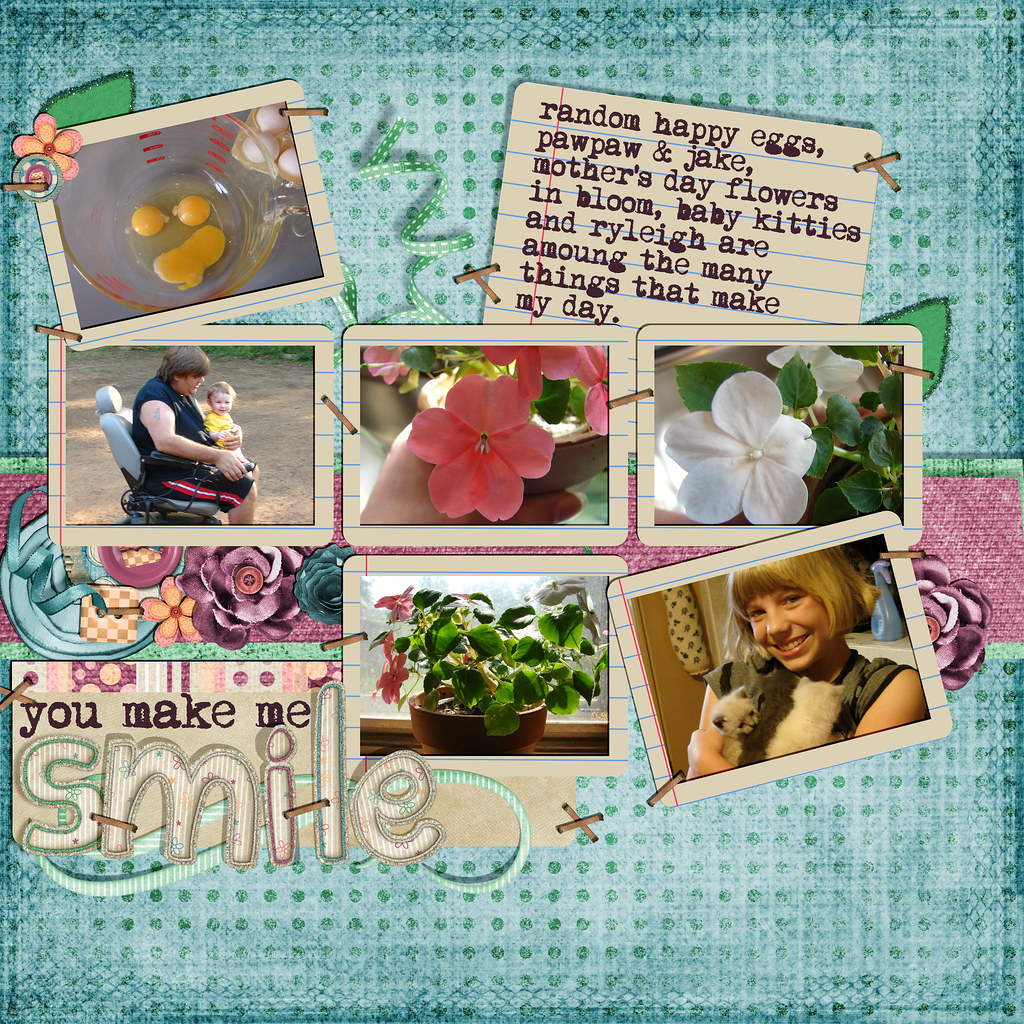This image depicts a detailed collage featuring six distinct photographs, all arranged on a visually engaging mixed media background with a teal hue and green polka dots. In the top left corner, a photo showcases eggs in a measuring cup, labeled "Random Happy Eggs". Adjacent to it, a man, presumably 'Paw Paw', is seen seated in a wheelchair holding a baby, presumably 'Jake', evoking a tender moment. Complementing these, the collage also includes images of vibrant pink and white flowers captioned "Mother's Day Flowers, In Bloom". Below these flowers, a bowl of assorted blossoms further enhances the floral theme. Central to the bottom section, a young woman with blonde hair joyfully smiles at the camera while holding two kittens, tagged as "Baby Kitties". The collage wraps up with the inspirational message "You make me smile" on the bottom left, featuring a creative 3D font. The entire composition, accentuated with a loose-leaf paper styled border, beautifully captures precious moments and elements that bring joy.